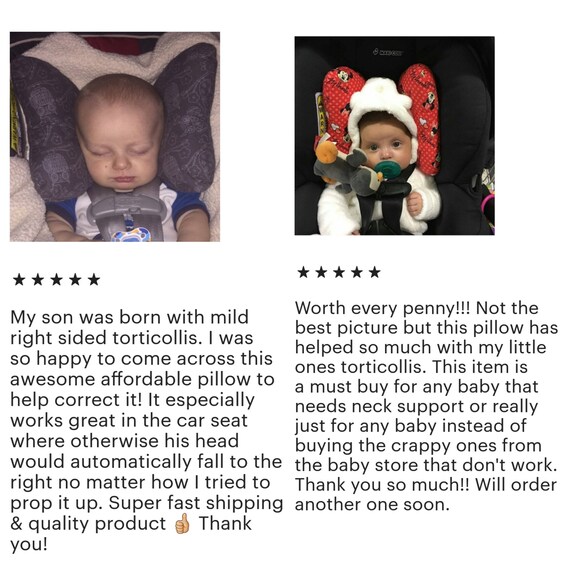The image features two detailed reviews for a baby neck support pillow designed to help with conditions like torticollis. On the left side, there is a photograph of a sleeping baby boy in a car seat. The baby wears a white shirt with blue sleeves and has a bit of blonde hair. His head rests on a gray, butterfly wing-shaped pillow, and behind him, there's the edge of a pink blanket. Below the picture, five black stars denote a five-star review. The accompanying text below praises the pillow for its affordability, effectiveness in aiding mild right-sided torticollis, and its suitability for use in a car seat, noting the fast shipping and high quality of the product.

To the right, there is another photograph of a baby in a black car seat. This baby is awake, wearing a white hat and clutching a gray penguin toy. The baby has a green pacifier and brown eyes, and is dressed in a white shirt. The baby's head is supported by a red, butterfly wing-shaped pillow, possibly with a Minnie Mouse or Mickey Mouse pattern. Like the first review, five black stars are displayed beneath the photo. The review text highlights the pillow's worth, affirming its effectiveness for babies needing neck support and particularly praising its utility in addressing torticollis. 

Overall, both reviews emphasize the pillow's benefits in providing neck support and correcting torticollis in infants, with particular praise for its performance in car seats and the overall quality and value of the product.